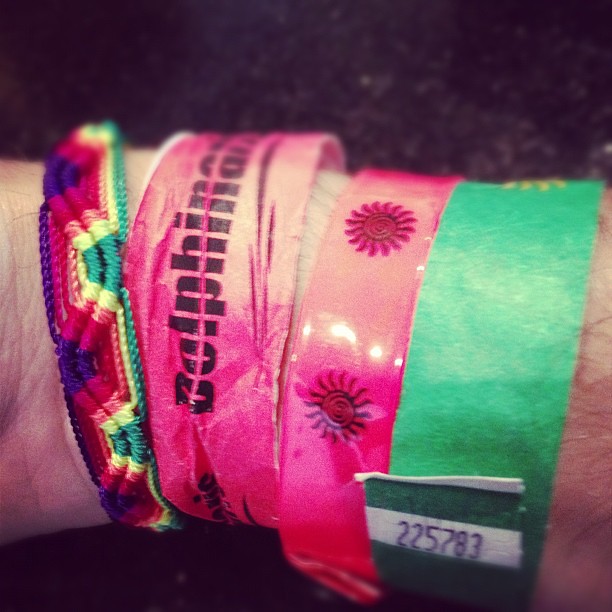In the photograph, you see a close-up of a hairy right wrist adorned with four distinct wristbands. The background is a muted black, possibly indicating an indoor setting and the use of a cell phone flash. Starting from the left, the first wristband is a handmade, embroidered friendship bracelet featuring a rainbow wave pattern with colors including purple, red, orange, yellow, and green. Next to it is a green Tyvek wristband with a partial view of yellow detailing on the left and a sequence of numbers partially visible, suggesting it might be from an event or festival. The third wristband is a pink plastic band adorned with Aztec-style sun designs in a darker hue. Finally, the fourth wristband is another pink Tyvek band, thicker than the others, bearing the text "DOLPHINA" in dark purple writing, although some of the text is obscured. The base of the thumb is visible on the left side of the image, adding a personal touch to this eclectic collection of wristbands.